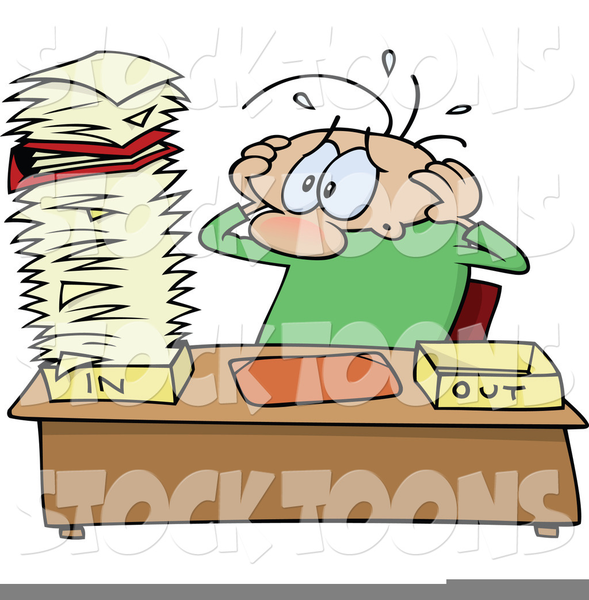In a simple, Kathy or Dilbert-like American cartoon style, the image features a presumably male character seated at a brown desk, conveying a sense of distress. The character, who has a few wisps of hair sticking out from his head, is depicted with large eyes, a large nose, and a green shirt. His eyebrows hang off the side of his football-shaped face as he clutches the sides of his head with his thin arms, having only three visible fingers on each hand. Sweat droplets can be seen popping off his head, emphasizing his overwhelmed state. In front of him, the desk showcases a towering pile of papers in the 'In' box, extending past his head, while the 'Out' box on the other side remains entirely empty. Adding to the humorous yet stressful scene, a transparent watermark with chunky, cartoonish font and drop shadow reading "StockTunes" is prominently repeated across the image.